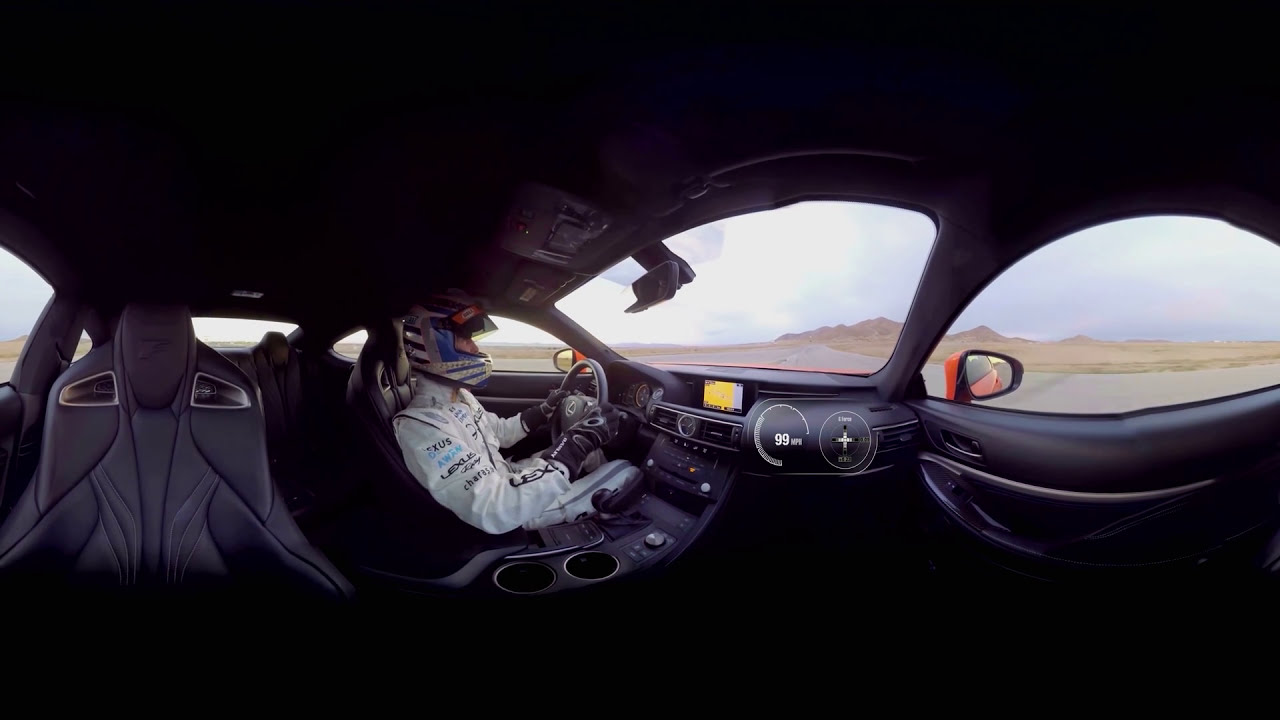In this image, we see the interior of a high-end Lexus vehicle, which appears to be a test car. At the center, a man dressed in a white jumpsuit emblazoned with the Lexus logo is seated in the driver's seat. He’s wearing a blue, white, and red helmet, along with black gloves, firmly grasping the steering wheel. The empty passenger seat and vacant cupholders are visible. The dashboard and console appear sleek, with yellow detailing on the console. 

The scene outside the car reveals a relatively cloudy day with a clear road ahead. Through the car windows, there is a small brown mountain range visible in the distance. This implies the setting is likely outdoors, presumably during a daytime test drive.